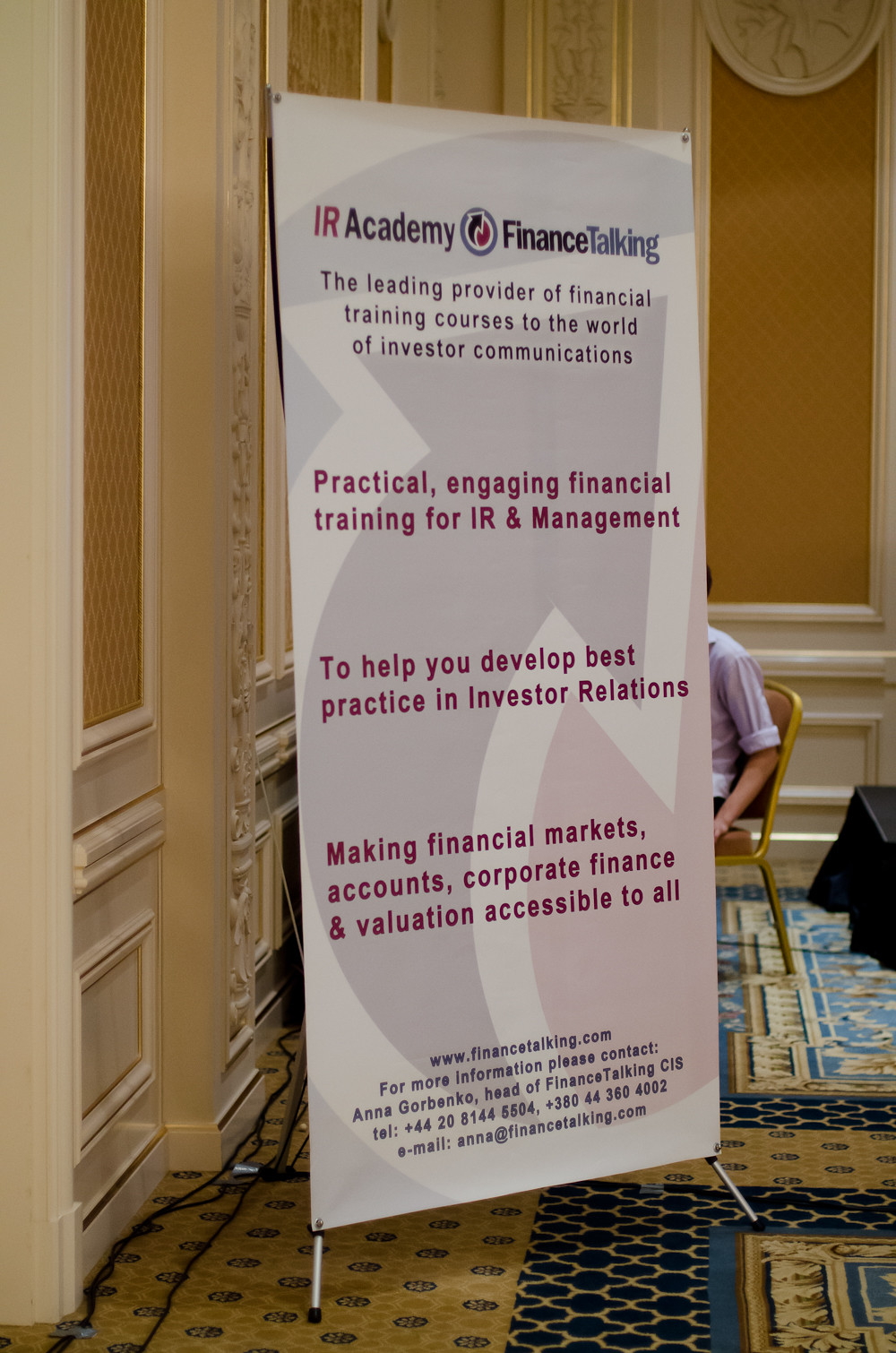The photograph showcases a tall, freestanding poster for the IR Academy, prominently positioned on the intricately designed, gold and blue carpeted floor of what appears to be a high-end hotel or convention center. The poster features a white background adorned with subtle, light-colored red and blue arrows pointing upwards and downwards. The header reads "IR Academy Finance Talking," proclaiming itself as the leading provider of financial training courses for the world of investor communications. The banner elaborates on offering practical and engaging financial training for investor relations (IR) and management, aimed at making financial markets, accounts, corporate finance, and valuation accessible to all.

The sign stands on metallic legs, and below the main text, it provides contact information: a website (www.financetalking.com), and details for Anna Gorbenko, Head of Finance Talking, including a couple of international phone numbers and an email address. The environment is further characterized by the hotel’s white and creamy yellow walls decorated with intricate patterns. Additionally, some electrical wires run along the carpet near the lower left side of the photograph. In the background, there is a seated individual whose shoulder and left arm are visible, hinting at a busy, professional setting, possibly in the midst of a conference or seminar.